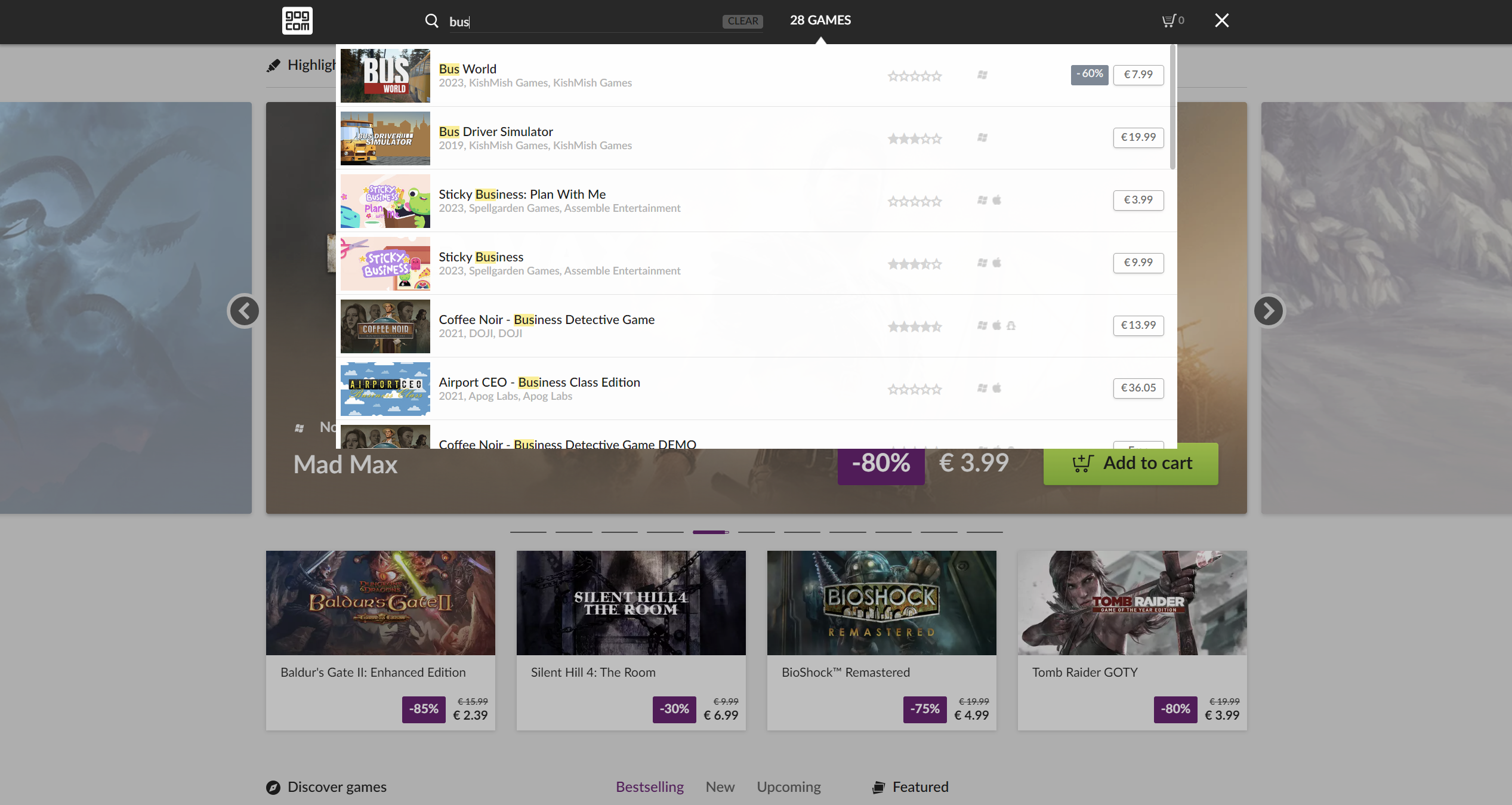The website interface has a sleek, black-themed design. On the left side of the header, there is a white square that appears to display the text "GOG.COM" in black. Adjacent to this is a white magnifying glass icon, indicating the search function.

When "B-U-S" is typed into the search bar, suggestions appear, each highlighted with a yellow marker around the word "bus." The first suggestion is "Bus World," a 2023 release by Kishmish Games, priced at €7.99. Following that is "Bus Driver Simulator," a 2019 game also by Kishmish Games, listed for €19.99.

Next up is "Sticky Business: Playing With Me," from 2023 by So Garden Games and Istanbul Entertainment, available for €3.99. Similarly, "Sticky Business" from 2023 by the same developers is priced at €9.99.

Further down, "Coffee Noir: Business Detective Game," a 2021 release by Doji, is available for €13.99. Lastly, "Airport CEO: Business Class Edition," from 2021 by APOG Labs, is listed at €36.05.